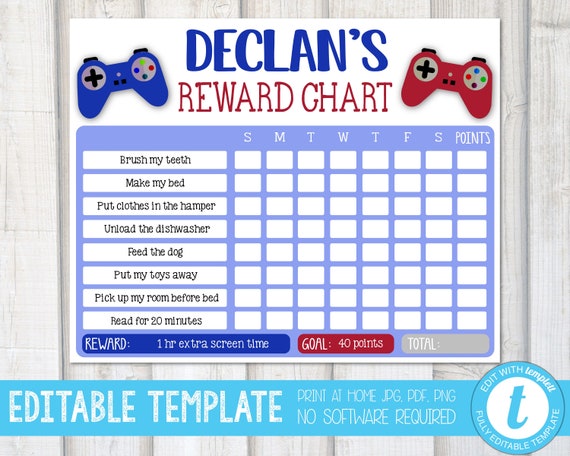The image titled "Declan's Reward Chart" features a detailed children's chore chart designed to incentivize good habits with extra screen time. Set against a gray wooden background, the chart's header is in blue text stating "Declan's," followed by "Reward Chart" in red. Flanking the chart are two cartoonish gaming controllers, a blue one on the left and a red one on the right.

The chart is organized with columns for each day of the week from Sunday to Saturday, alongside a final column for tallying points. Listed chores include: brush my teeth, make my bed, put clothes in the hamper, unload the dishwasher, read, feed the dog, put my toys away, pick up my room before bed, and read for 20 minutes. Accumulating 40 points grants Declan one extra hour of screen time. 

At the chart's bottom, the text specifies that it is an editable template, printable at home in JPG, PDF, or PNG formats, with no software required. A small logo featuring the letter 'T' accompanies this description. The overall design looks like an image from a web catalog or advertisement promoting this customizable reward chart template.